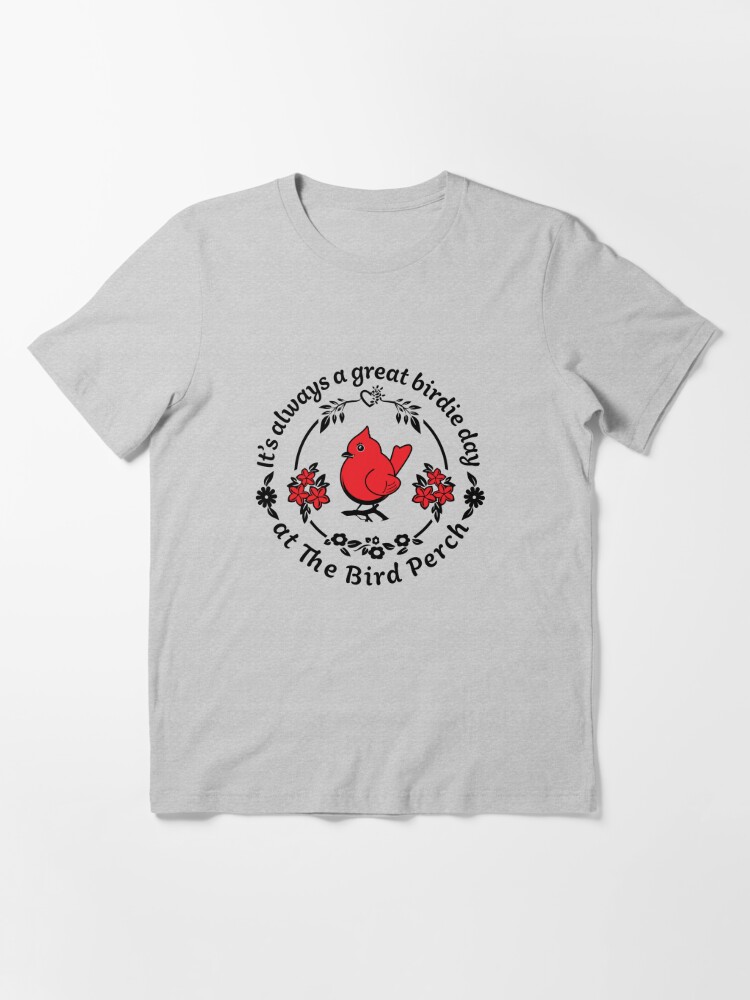This image portrays a short-sleeved gray t-shirt, laid flat against a white background, with no one wearing it, typical of a product listing photo on an online store. The shirt features a central design that encapsulates a cheerful message about birdwatching. Dominating the middle of the t-shirt is a red cardinal, which serves as the focal point of the entire design. Surrounding the bird is a smaller circle that has two sets of three red flowers on either side of the cardinal. Encircling this inner motif is a larger circle bearing the text, "It's always a great birdie day at the bird perch," written in black, with the top part of the phrase arching over the cardinal and the bottom part curving underneath. Complementing this, there are small black flower doodles positioned on both the right and left sides of the larger circle. The shirt itself appears suited for children, teenagers, or small adults, and might be particularly appealing to females. The simple yet engaging design combines the charm of a red cardinal and floral elements with a playful, circular text layout, making it a delightful garment for nature enthusiasts.